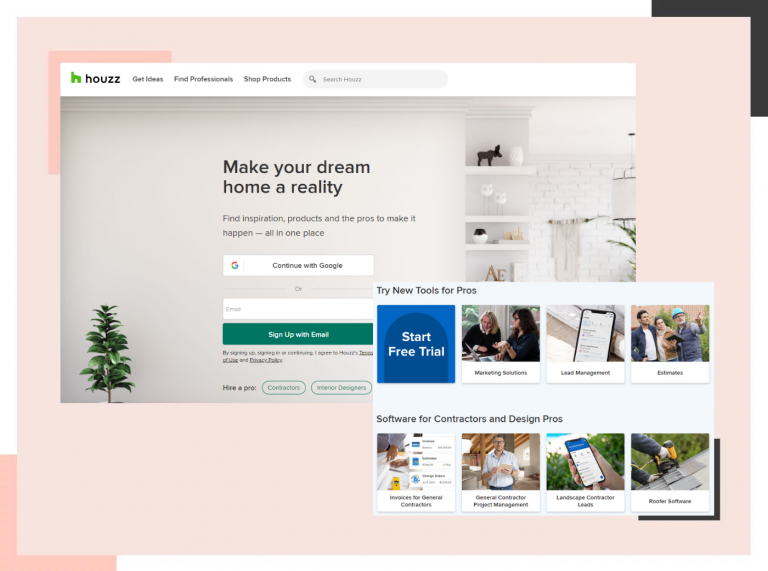The image depicts a website interface with a predominantly light pink background. The design is framed by a black border in the upper right-hand corner and a slightly darker pink border in the lower left-hand corner, resembling the corners of a picture frame.

Within this frame, the central content is highlighted by a white banner featuring a search bar. The banner includes the brand name "H-House" and navigational options such as "Get Ideas," "Find Professionals," and "Shop Products." Below the search bar, a prompt reads, "Make Your Dream Home a Reality. Find inspiration, products, and the pros to make it happen all in one place."

For user access, there are options to "Continue with Google" or "Sign in with your email." The backdrop presents a minimalistic white wall adorned with a small green tree on the left and some curios on a cabinet. Behind this scene, a fancy white curtain with wind chimes is faintly visible. 

Additionally, an inset image promotes tools for professionals, accompanied by text encouraging users to "Try New Tools for Pros," highlighting offerings like free trials and contractor software specifically designed for professionals in contracting and design.